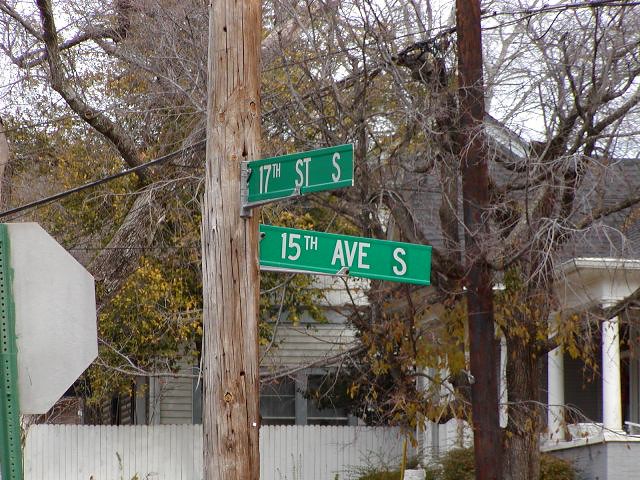This photograph captures a detailed outdoor suburban street scene, prominently featuring a wooden utility pole with green street signs for 17th Street S and 15th Avenue S, displaying white capital letters. Adjacent to this pole, there is a green post, upon which the back of a white octagonal stop sign is visible. The scene is set in front of an average-sized white house with a black roof and a patio entrance accented by columns. However, much of the house is obscured by trees, one of which is still adorned with leaves while the other is nearly bare. A white picket fence runs along the front of the property, adding a charming touch to the scene. The complex layering of elements—including the utility poles, street signs, trees, and partially visible house—creates a rich, textured tableau of suburban life.